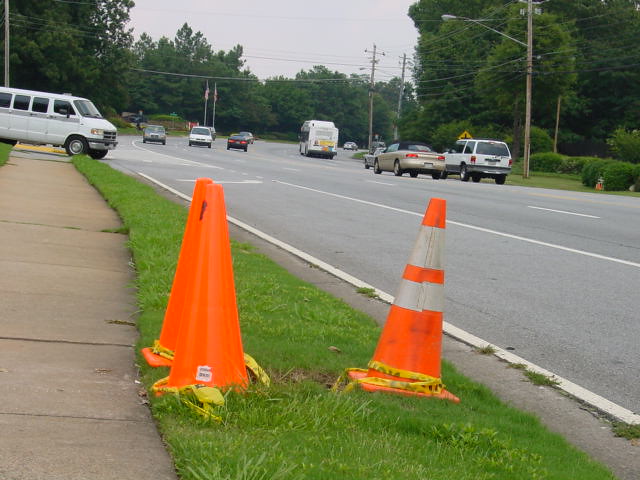The photograph captures a roadside scene from the perspective of a sidewalk situated adjacent to the road. Prominently in the foreground, a well-manicured strip of green grass separates the sidewalk from the road. Positioned amidst the grass are three traffic cones encircling an indistinguishable object. To the left of this area lies another stretch of sidewalk. In the mid-background, there is a junction where a street intersects with the main road, and a van is stationed at this point, seemingly poised to turn but currently idle.

The main road itself comprises two lanes in each direction, accompanied by a central turn lane, and contains moderate traffic moving both ways. Further into the background, a dense canopy of trees provides a lush, verdant backcloth. Overhead, a network of telecommunication or power lines supported by tall utility poles spans the scene, contributing to the urban infrastructure. The photograph is set against an overcast sky, emphasizing the vibrance of the green grass and adding a moody ambiance to the image.